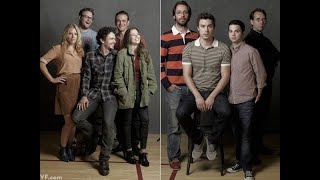The photograph features two separate group portraits divided by a central white line, with black bars running down the far edges. Each group stands against a gray background reminiscent of a gymnasium, identifiable by the wooden floor with red markings similar to a basketball court. The left image displays five young adults: a seated man with short black curly hair who is smiling, a blonde woman standing to his left, and another woman to his right wearing a green army jacket and black pants. Standing behind them are two men, both smiling. The overlay in the bottom left corner reads "vf.com." In contrast, the right image showcases four young men in casual attire. One man in the back dons a red and blue striped shirt with glasses, while the others are dressed in a mix of polos, a purple button-down, and a black outfit. Each individual in the group on the right appears to be looking directly at the camera with neutral expressions. Together, these images suggest a cast photo for a TV show or movie, highlighting a diverse collection of young adults in a relaxed setting.